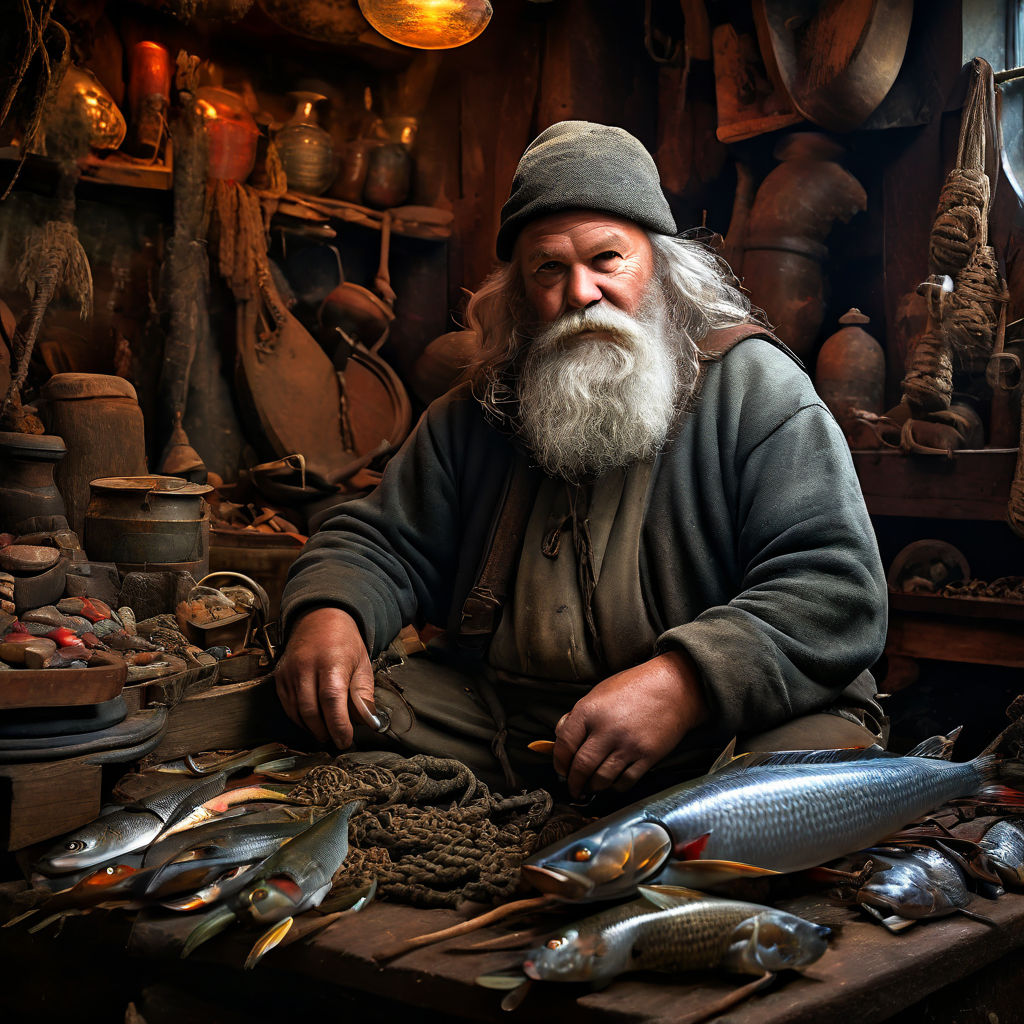The image depicts an elderly fisherman, likely in his 60s, with a long, flowing gray beard and hair that extends from under a gray, felt-like beanie. He appears rugged and muscular, dressed in layered clothing which includes a gray sweater, a light gray undershirt, and brown overalls held up by one suspender and a belt. His khaki-like pants complete his practical ensemble. The fisherman is seated at a cluttered workbench, surrounded by a mélange of fish, long and silver with varied fins, some possibly being used for bait. He diligently works with his hands, possibly preparing fishing nets or tackle, and holds a hook, indicating his trade. The setting is rustic and well-worn, with an assortment of metal and leather accessories, ropes, candles, a lantern, clay and wooden pots, and a pile of rocks around him, emphasizing a life intertwined with the sea and fishing. The overall scene has a timeless, almost AI-generated realistic quality, giving it a distinct, aged photographic feel.